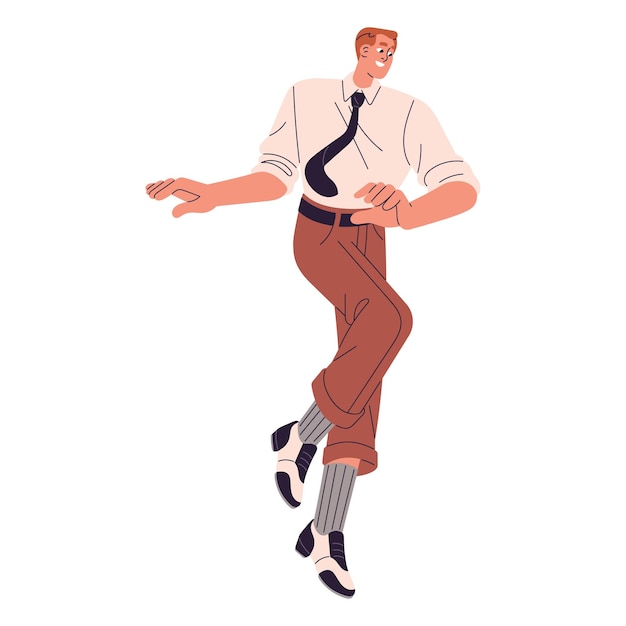This is a vibrant cartoon or animation drawing of a man dancing, rendered in a popular illustrated style known for exaggerated proportions and minimal border lines, often associated with Facebook corporate art. The man appears extraordinarily tall, possibly around 8 feet, with a comically tiny head that starkly contrasts his elongated, distorted body. He has short red hair and is smiling, looking off to the side. Dressed in a white long-sleeve shirt paired with a black tie, his ensemble also includes tan-colored pants with a black belt. The pants are rolled up once, revealing gray socks and white shoes with black markings on the tongue, heel, and toe. His dance pose is evident: one knee is lifted while the other foot is poised on its toes, with arms crooked at the elbows. This dynamic imagery is set against a clean, white background.